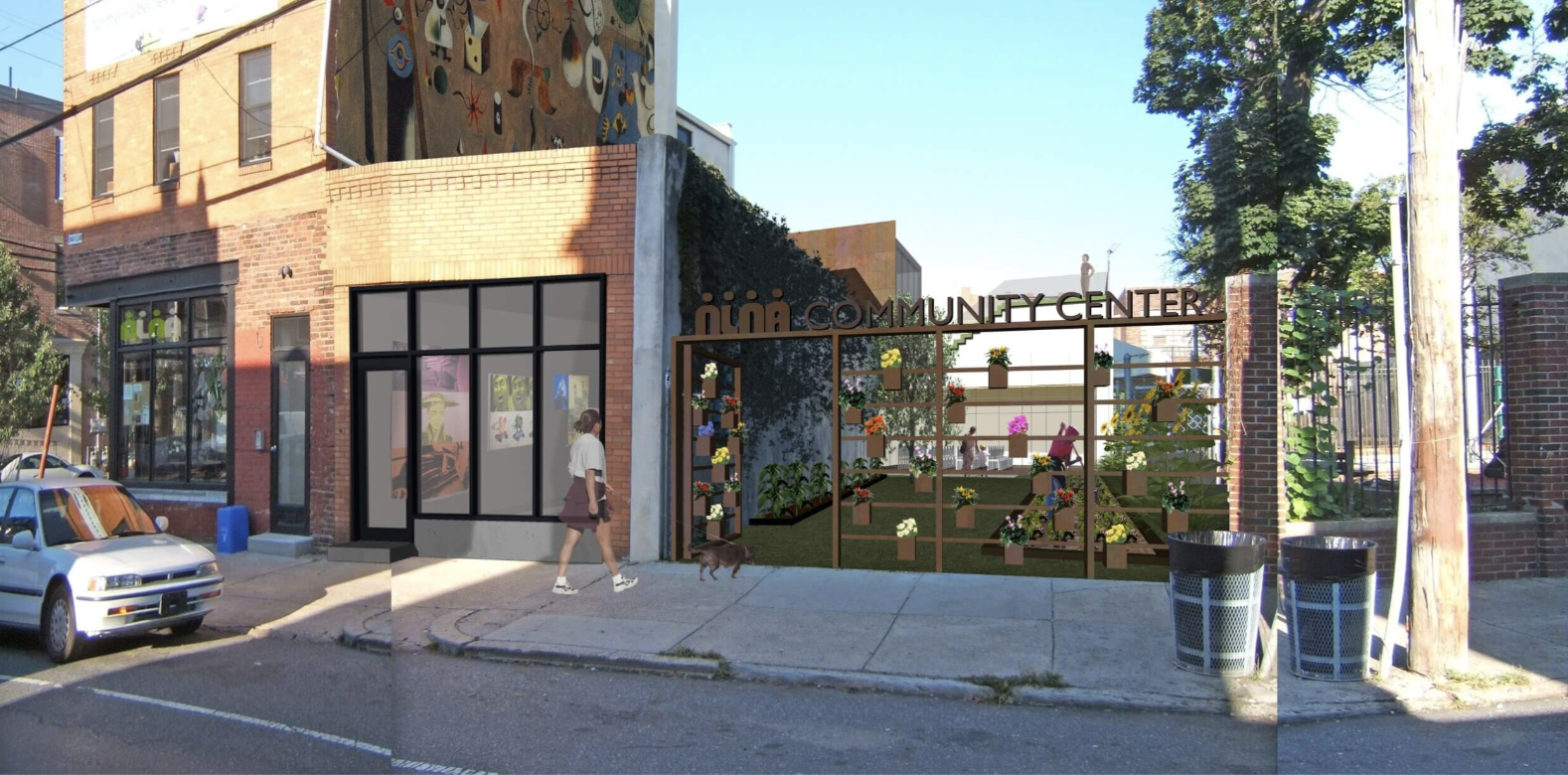In this screenshot from a video game, we see a detailed urban scene featuring a small, well-kept dog park labeled as the NLNA Community Center. Positioned between two buildings in a small city street, the park is adjacent to a brick music store, identifiable by the musical notes drawn on its façade. The store has black window frames on the first floor, with ivy cascading down its side and graffiti adorning the second floor. A light blue four-door sedan is parked at the curb, which shows signs of deterioration with grass growing through the cracks. The entrance to the dog park is marked by a metal gate adorned with planters and plants, and a sign that reads "NLNA Community Center." Inside, there's a neatly maintained garden. Nearby, two trash cans and a telephone pole can be spotted at the bottom right corner of the image. A woman is seen walking her dog into the park, under a clear, blue sky with noticeable evening shadows, suggesting the time is late in the day. The entire scene is bathed in a warm, peaceful atmosphere, reflecting the charm and community spirit of the neighborhood.